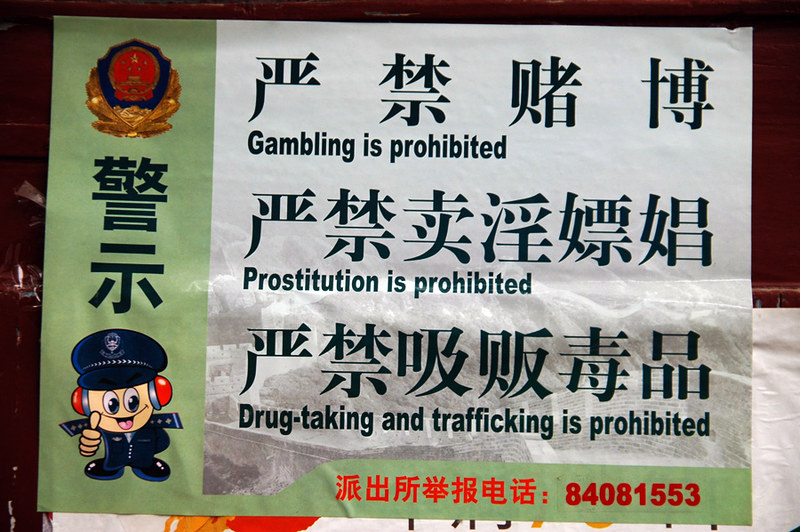The image depicts a sign prominently featuring prohibitions against gambling, prostitution, and drug taking and trafficking, conveyed in both English and Asian characters, likely either Korean, Chinese, or Japanese. The sign appears to be possibly suspended from a ceiling, with an indeterminate background. On the far left, a green vertical strip runs the length of the sign, topped by a distinctive emblem comprising a blue and gold boundary encircling a red shield. Below this emblem, there are Asian symbols followed by an engaging cartoon image of a police officer. The officer sports a blue uniform with stars, a pilot's or flight attendant's hat bearing an insignia, and wears what resemble red sirens on his ears; he smiles with wide, oval eyes and gives a thumbs up. The right-hand side of the sign features a white section with black text displaying "Gambling is prohibited," "Prostitution is prohibited," and "Drug taking and trafficking is prohibited," each interspersed with additional Asian characters. On the bottom left, the green strip continues with more Asian symbols and the red number "8408-1553" on an olive background, framed by what may be an orange or green border. The varied text and elements suggest a public notice or warning likely found in an Asian country.